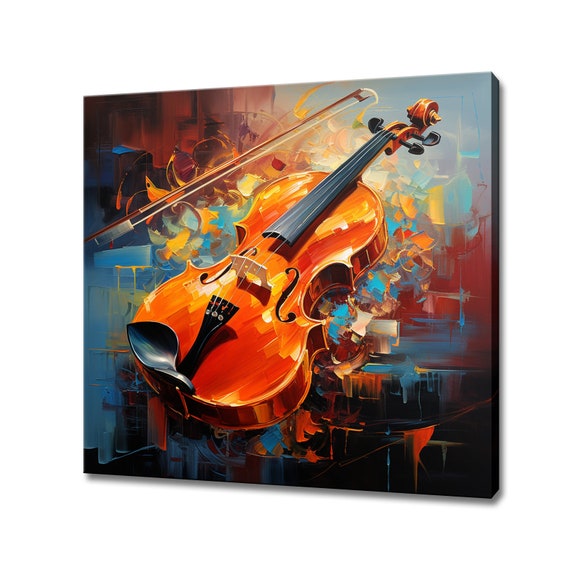This vibrant and colorful painting prominently features a violin and a violin bow, rendered in a rich orange wood color with striking black details. The violin sits centrally in the composition, standing out against an intricate, abstract background. The backdrop is a dynamic blend of shades, including bright yellows, oranges, blues, pinks, and blacks, creating a sense of movement and depth. Haphazardly scraped paint and abstract patterns suggest a cityscape or shifting forms, with square patterns and melting brush strokes adding texture. The colors are brighter and lighter at the top, transitioning to darker hues at the bottom, enhancing the overall visual impact. This captivating piece of art would undoubtedly appeal to both musicians and art lovers alike.